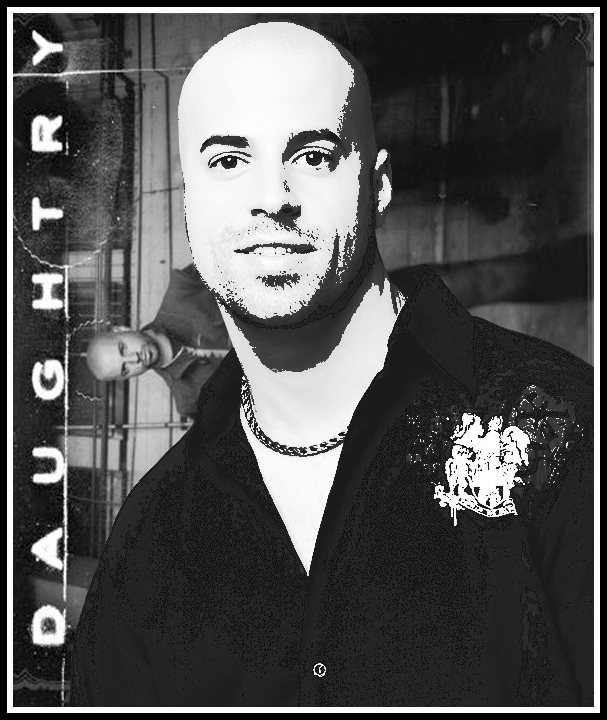This black and white photograph features a bald white man identified as Chris Daughtry. He has a distinct set of dark eyebrows, a bit of a mustache, and a beard. Daughtry is seen wearing an unbuttoned black collared shirt with a gold chain necklace around his neck. A white and black graphic insignia is noticeable on the upper left side of his shirt. The image has a high contrast, making his facial features and the shadow on the right side of his head particularly prominent. 

In the background, a secondary image of Daughtry is rotated 90 degrees counterclockwise, showing him in a black jacket and extending out from the neck of the primary foreground image. This background figure also appears bald and is gazing directly at the camera, mimicking the main image's orientation but turned sideways. The entire composition gives a surreal, layered appearance, enhanced by the overexposed quality of the photograph.

On the left side of the image, the name "Daughtry" is written vertically in white font, with the letters running from the bottom left to the top left, reinforcing the graphic design's textural complexity.